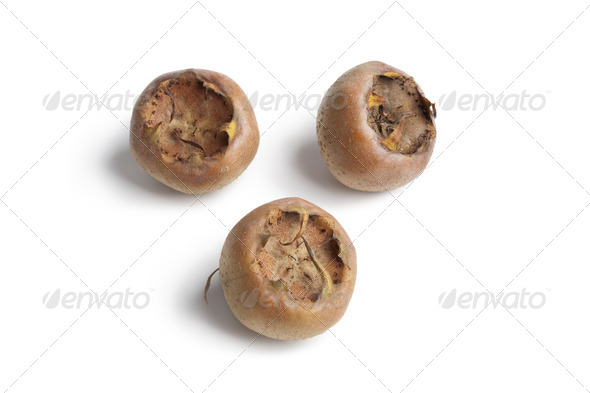The image showcases three brownish, spherical objects resembling nuts or seed pods, arranged in a triangular formation with two at the top and one at the bottom. These objects feature slightly hollowed centers, varying in shades from light to medium brown, with some hints of darker and softer textures within the hollows. The background is marked by a patterned grid of thin, diagonal lines creating diamond shapes, and is watermarked multiple times with the text "Envato" and an accompanying leaf logo, providing a protective overlay across the image. The overall setting combines the tactile contrast of the objects with the structured complexity of the background.